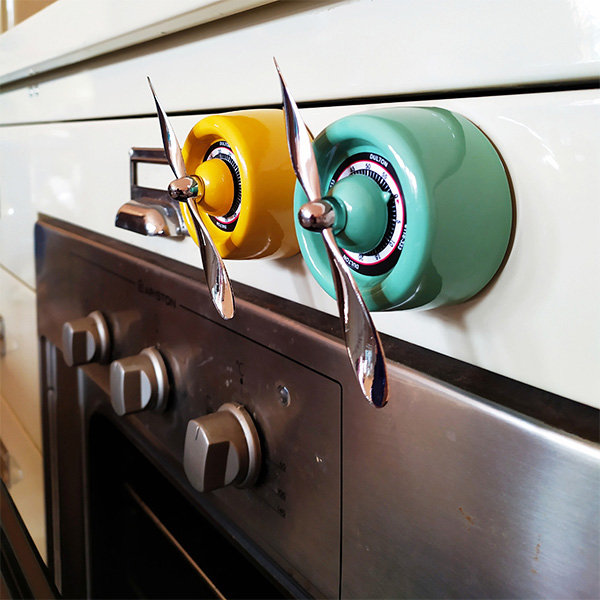This photograph captures a curious and somewhat perplexing kitchen scene centered around a brushed stainless steel oven embedded in a white, glossy cabinet. At the forefront of the image is the oven door, featuring several stainless steel control knobs along the top edge. Directly above the oven, dominating the picture, are two peculiar and eye-catching kitchen timers. Each timer is cylinder-shaped: the left one in a vibrant yellow and the right one in a bright teal. These timers have circular faces with numbers, possibly for setting durations, and are topped with stainless steel propeller-like mechanisms that are similar to miniature airplane propellers. These propellers extend roughly 50% wider than the body of their respective cylinders. Above these avant-garde timers is a simple stainless steel drawer handle, completing the unusual array of elements in this modern kitchen appliance composition.